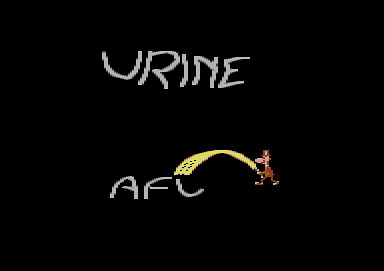The image features a completely black background with digitally created text in the center. Approximately two inches from the top, the text displays the letters "U," "R," "I," "N," and "E." The "U" resembles an excessively wide and slightly curved "V," while the other letters vary in size and alignment, with the "N" being barely legible and the "R" and "E" appearing oversized and misaligned. About two inches below this text, in gray, are the letters "A," "F," and "C." At the top of the "C," there is a 3D rainbow-like arc in yellow, which extends back to touch a small brown figure. The figure features a light brown snout and a black nose, gripping the yellow arc as if holding it.